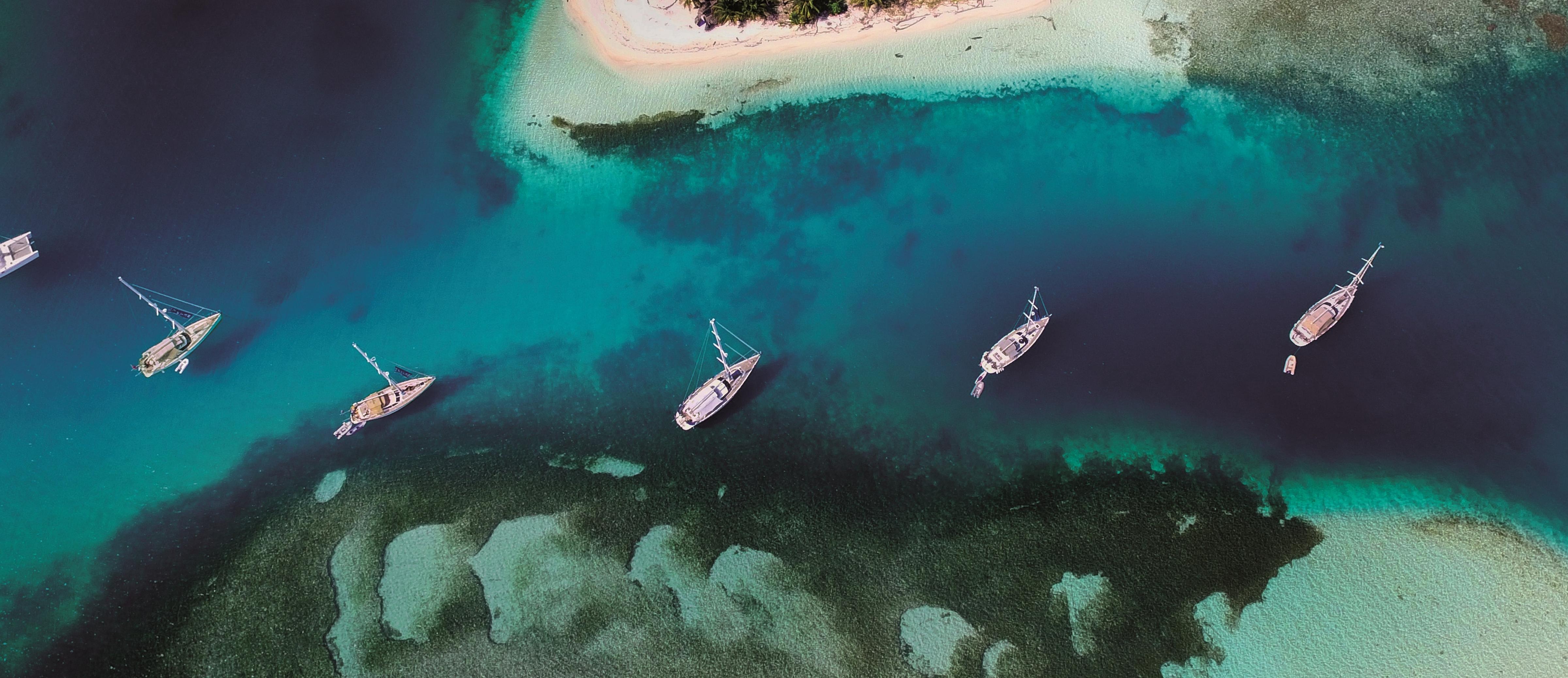This aerial photo, likely captured by a drone or plane, showcases a serene scene of a crystal blue inlet with six white boats featuring large masts and sails, which are currently not raised. These boats are arranged diagonally across the middle of the image, resting in a clear turquoise and deep teal channel. The water's transparency reveals underlying algae and aquatic plants. The bottom half of the picture displays a small shoreline dotted with patches of white sand, pale tan rock outcrops, and scattered greenery, possibly seaweed or moss. The top of the image mirrors this with another white sandy shoreline adorned with hints of greenery, suggesting a landmass or island. The boats, with their distinctive unraised sails and uniformly white bodies, create a peaceful yet dynamic element against the backdrop of vibrant, gradated blues of the sea.